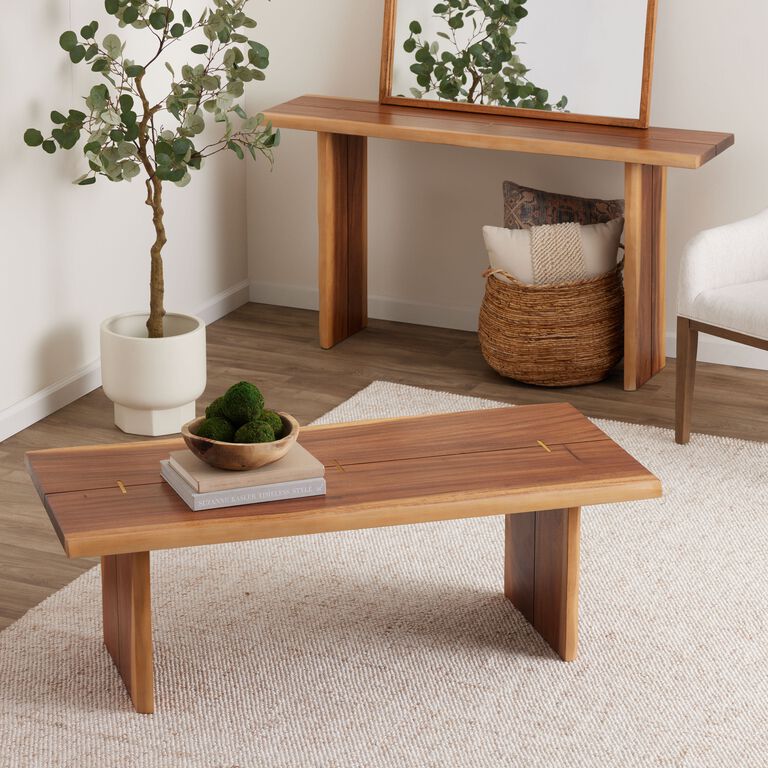The scene captures a cozy corner of an Asian-styled living room featuring a variety of wooden furniture elements set against a wood-seamed floor that is mostly covered by a thick, off-white carpet. In the foreground, there is a wooden bench that holds a bowl with a collection of greenish, earthy-looking balls atop two stacked books. Directly behind the bench stands a white floor vase with a small tree growing out of it, extending a hint of nature into the space. Adjacent to the tree, a wooden side table that mirrors the bench's design holds up a mirror that reflects the leafy branches. Beneath the table is a basket with a couple of pillows peeking out. To the far right of the image, partially captured, is a white chair supported by wooden legs. The overall aesthetic is reminiscent of an Ikea showroom, marrying functionality with minimalist design.